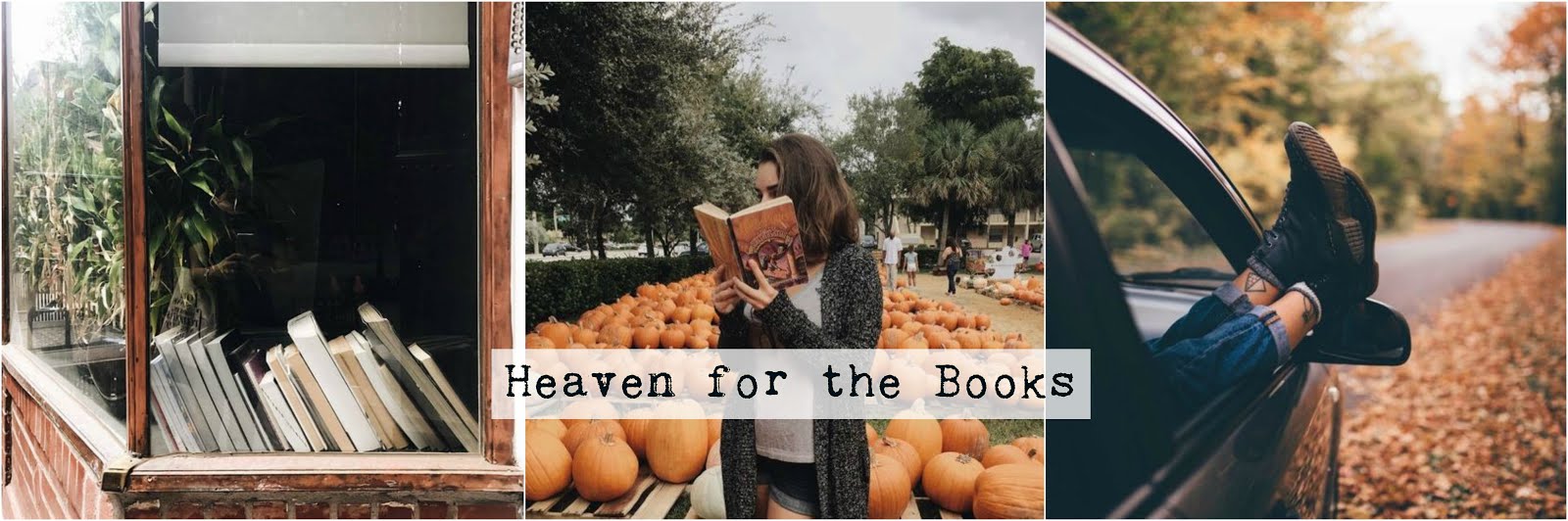This is a three-photo panel in portrait orientation, containing three square images aligned horizontally. The leftmost photo depicts a rustic, raw-hewn wooden shelf set against a backdrop of trees and sky. The shelf, resting on a brick wall, holds a disarrayed collection of thin old books laid horizontally with their spines facing upwards. The interior of the shelf is painted black, enhancing the contrast with the vibrant outdoor setting. The central image features a young Caucasian woman with long, dark brown hair, obscured partially by a book held up to her face with both hands, suggesting she is engrossed in reading. She is dressed in a gray or black cardigan over a white sweater and dark jeans and is standing amidst an expansive pumpkin patch, surrounded by numerous bright orange pumpkins. The background displays heavily canopied green trees against a clear blue sky. A transparent white bar with black lettering reading "Heaven For Books" stretches horizontally near the bottom of this photograph. The rightmost image shows a close-up of a pair of legs in blue jeans, with feet in black sneakers sticking out of a car window at a diagonal. The car, partly visible and likely red or brown, is positioned on a road strewn with orange autumn leaves, flanked by trees exhibiting a mix of green, yellow, and orange leaves. The upper right corner shows a clear blue sky, completing the outdoor autumnal scene. Across all three images, a white horizontal band with black text at the bottom center reads, "Heaven For Books."